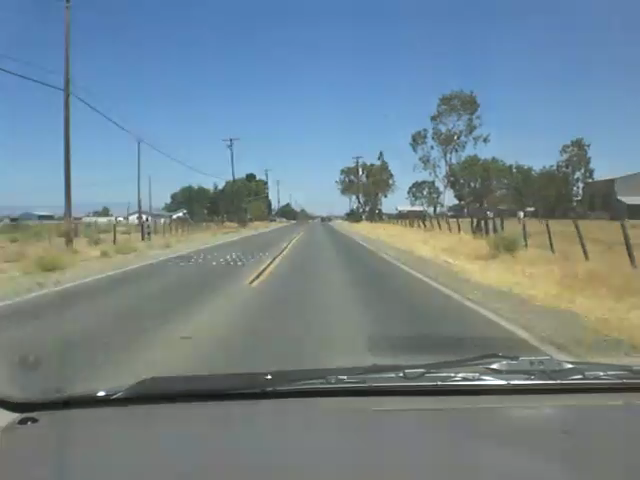The photograph, a somewhat pixelated color image, is taken from inside a vehicle through the windshield. The bottom third of the image displays the vehicle's grey and black dashboard along with a windshield wiper crossing horizontally. The road ahead is devoid of any other vehicles and features a double yellow line in the center and solid white lines marking the edges. On the right side, the road is bordered by a yellowish scrubland with sparse green bushes, stretching into a bank. Similarly, the left side of the road is flanked by dry, straw-like grass and low green bushes.

In the far distance, there are green trees, along with telegraph poles to the left, stringing power lines parallel to the roadway. Fences, simple and made of basic wooden posts and wire, align on either side. Further on the left, the photograph captures some low barns, contrasting with taller structures or possibly barns on the right.

The sky is a brilliant, clear blue, providing a sharp backdrop to the scrubland. The image resolution deteriorates towards the edges, making distant elements appear highly pixelated. The overall scenery stretches out towards the horizon, giving a feeling of endless travel through a sparse, somewhat desert-like landscape.